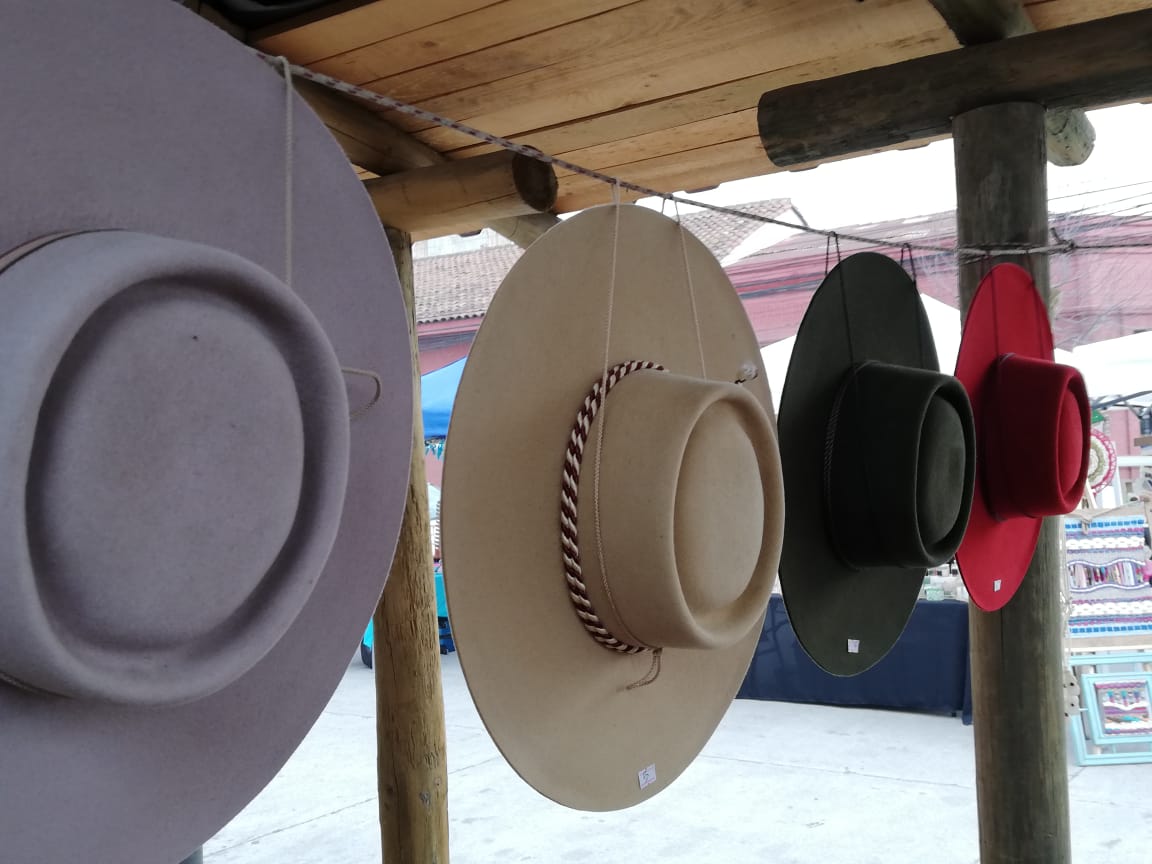This photograph captures an outdoor daytime scene at a small sidewalk shop or stand, likely part of a flea market, yard sale, or fair. The stand features a rough wooden slat roof supported by T-shaped wooden poles. Across the top of the image, a rope is strung from which four wide-brimmed hats with flat tops hang. The hats, likely made from rawhide or similar material, are arranged in the following order: a purple hat, a tan hat with a brown and white band around its middle, a black hat, and a red hat. Each hat appears to have a small price tag attached. In the background, other structures, possibly selling additional items such as art, and parts of a building or house with covered areas, are visible. The perspective is angled, giving an eye-level view of the hats and emphasizing their display.